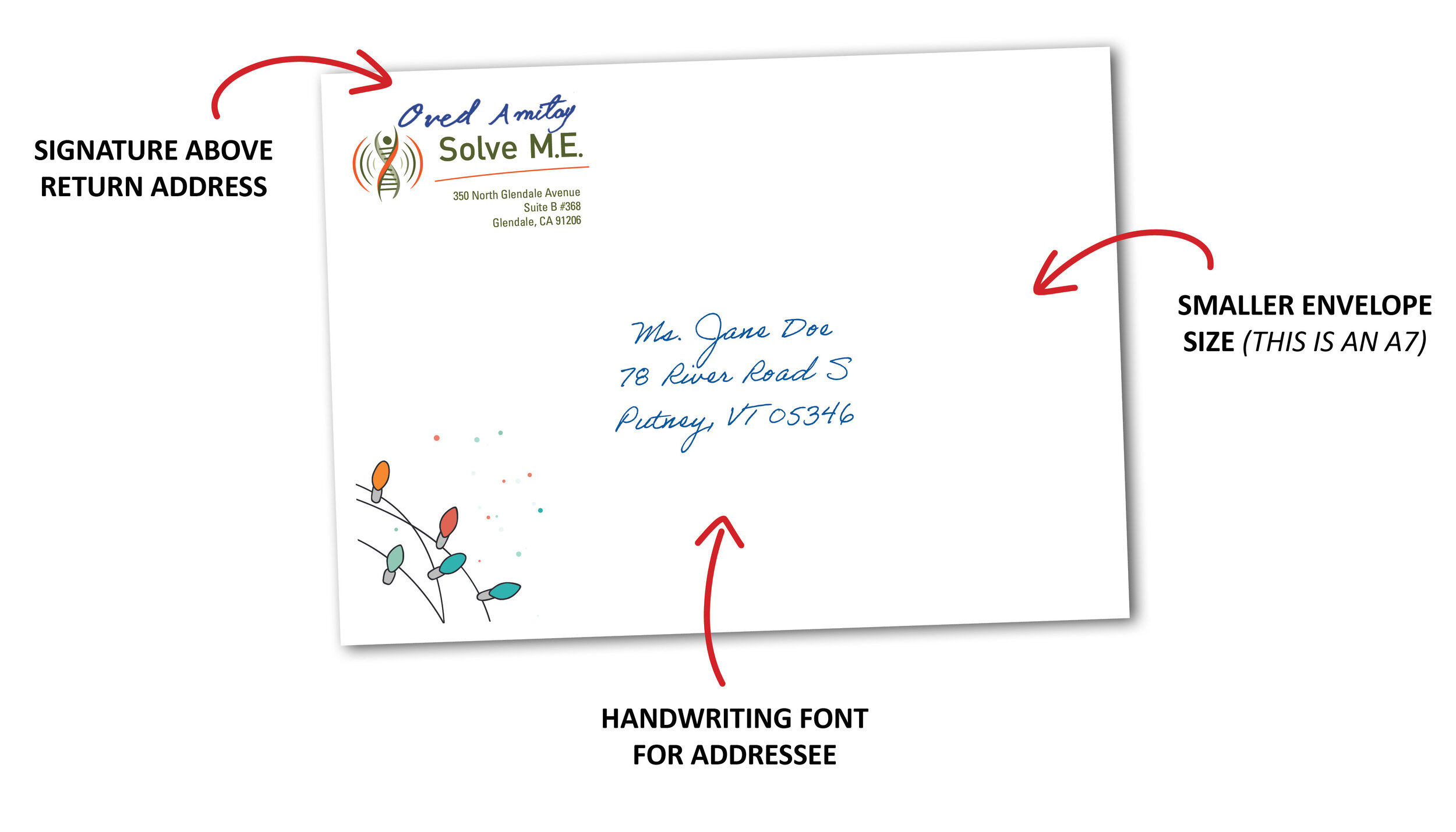The image is a detailed instructional guide on how to address an envelope. The letter has a white background with a Christmas or holiday theme accentuated by colorful ornaments in the bottom-left corner. These ornaments are colored orange, red, blue, turquoise, and cyan, and are grouped together with black strings, emitting a faint hint of color.

On the top-left corner of the image, arrows and labels guide the viewer on where to place important elements. A red arrow points to the top-left section that reads "signature above the return address." Here, an example shows a blue signature above a green return address labeled "Miss Jane Doe" with an address in Vermont, written in blue cursive font.

In the middle, the text directs attention to the "handwriting font for addressee." This area illustrates in blue cursive handwriting, with the address ending in the postal code "05346."

Finally, the right side of the image specifies the envelope size, indicating that it is an A7 envelope. This comprehensive visual guide ensures that the envelope is correctly formatted, highlighting where to place the return address, the recipient's address, and signature, making the correspondence both functional and personable.